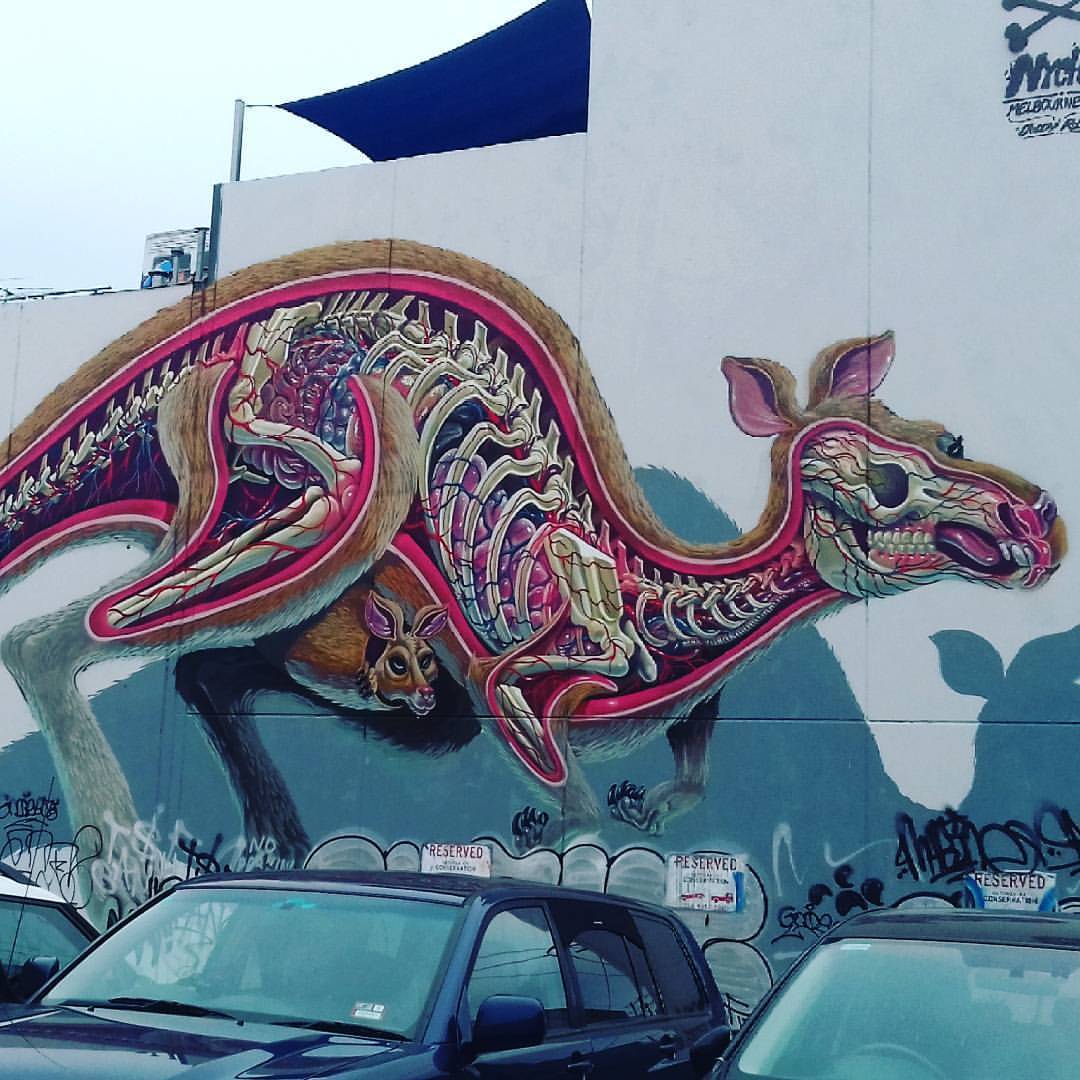The photograph captures a detailed and striking mural painted on a light blue wall, likely located in Melbourne, Australia, as suggested by the barely visible lettering in the top right corner of the image. The mural depicts a giant kangaroo, partially anatomically dissected, showcasing the intricate details of its internal structures such as the skeletal system, including the vertebrae, spine, rib cage, and leg bones. The kangaroo is also carrying a joey in its pouch, which remains intact and uncut. The mural, which feels reminiscent of a biology class illustration, shows the kangaroo with brown fur and appears slightly bent over with its front legs curled up. In the foreground, there are three cars parked in front of the mural, with "RESERVED" parking signs and tow truck imagery indicating these spots are designated.